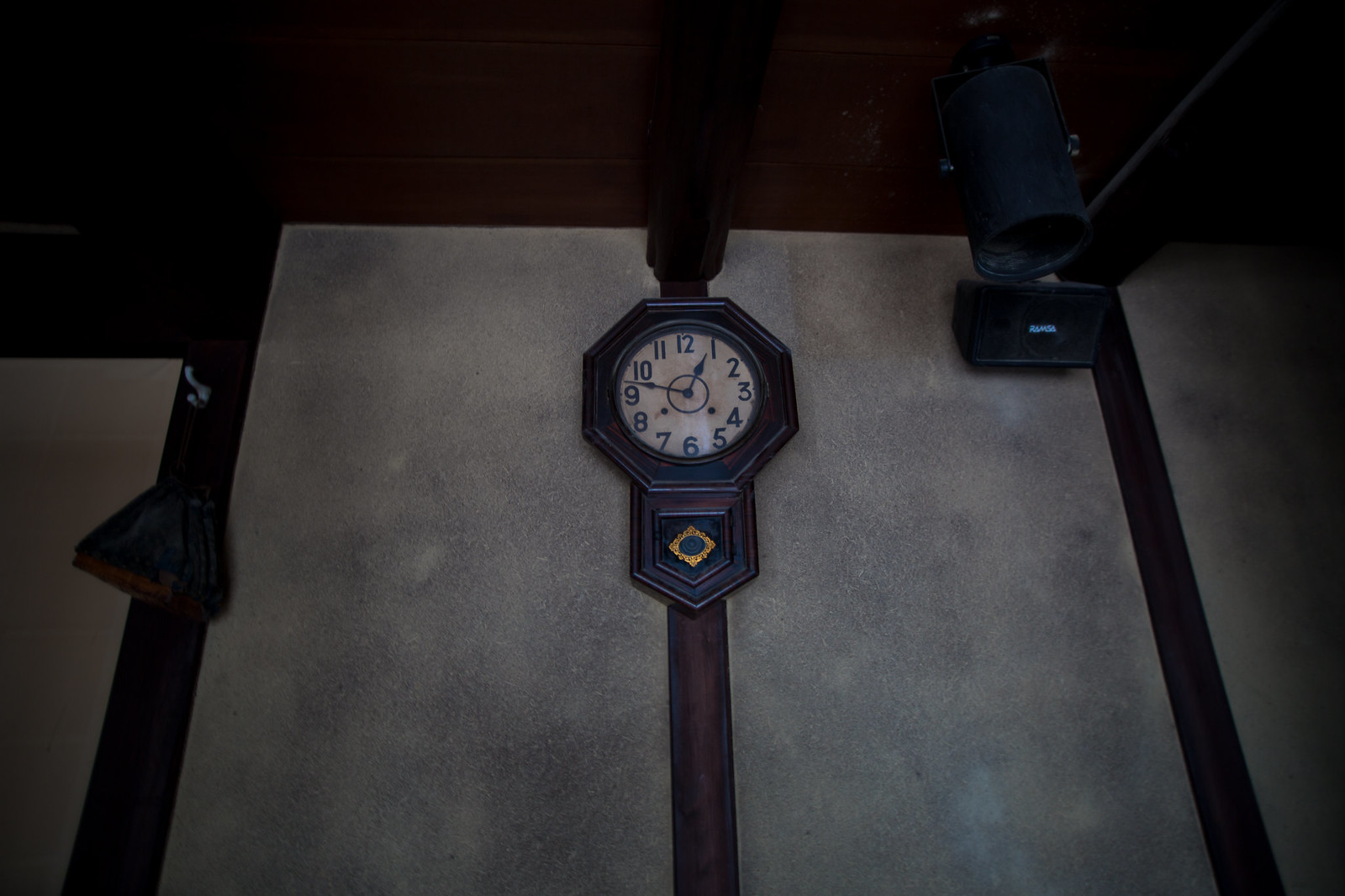This image captures a vintage small wall clock viewed from below, reminiscent of a grandfather clock design. The clock features an elegant octagonal face crafted from dark wood, offering a rich, timeless appearance. At the heart of the clock sits a dial with a weathered, brownish-white finish, lending an antique aesthetic. Bold black numerals encircle the face, clearly marking the hours. The clock's hour and minute hands are distinctively designed with spade-shaped ends; the minute hand extends further than the hour hand. The clock indicates the time as 12:49.

Directly beneath the octagonal face, a pointed rectangular wooden feature draws the eye. It houses a central bell, enhancing the clock’s traditional charm. This entire masterpiece hangs against a wooden wall plank that complements its dark wood hues.

Flanking the wooden plank, the wall is painted in a smoky gray shade, providing a subtle contrast that enhances the clock's prominence. To the right, a spotlight-style light fixture dangles from the wooden ceiling, casting a warm glow on the scene. Additionally, a rectangular speaker with a notably wide back is mounted in the upper right corner, angled downwards towards the floor, completing the quaint yet sophisticated setting.